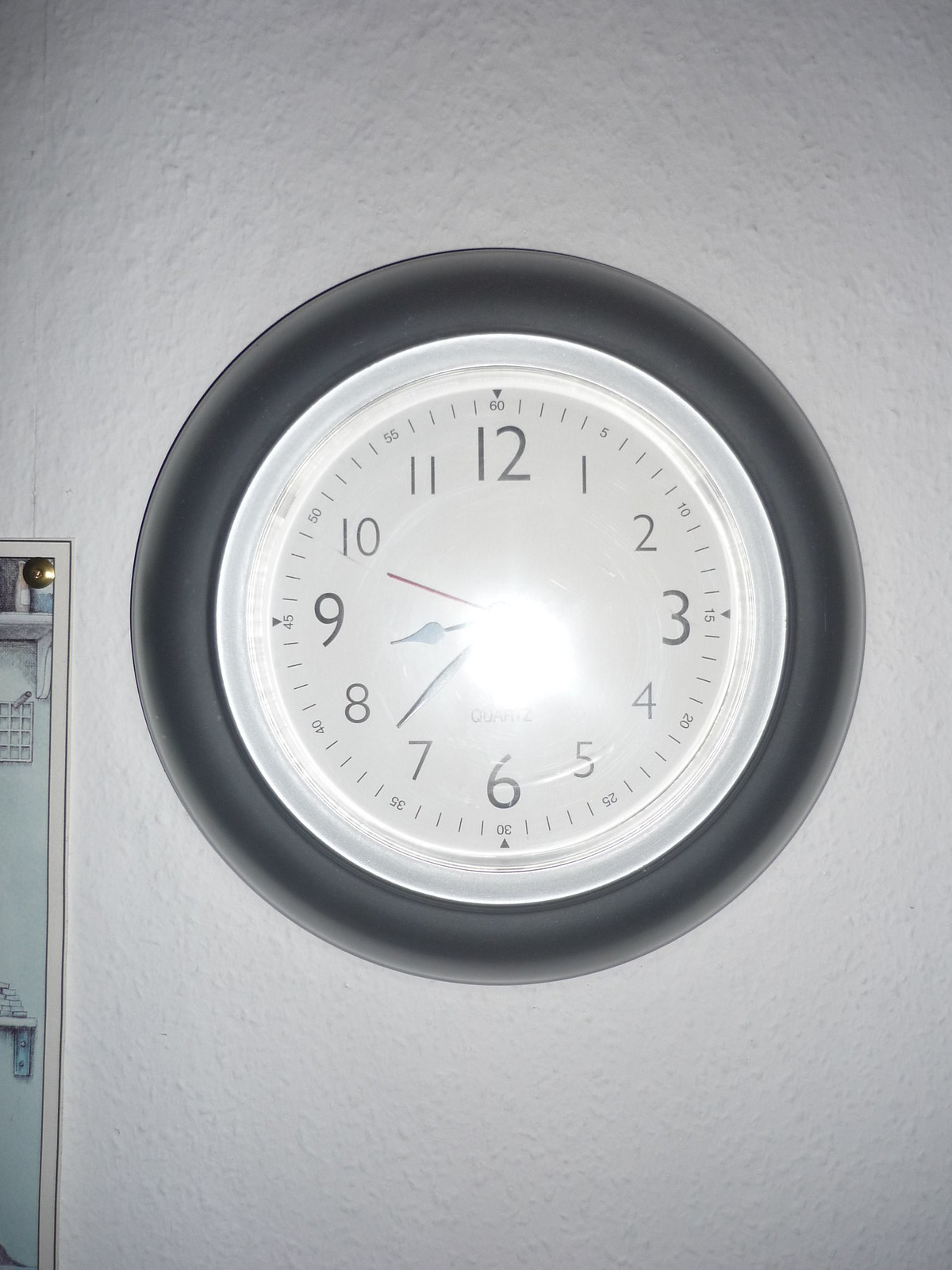This black-and-white photograph features an analog clock prominently mounted on a light gray wall. The clock is round with a dark gray outer rim and a very light gray face, possibly indicating a glass surface due to visible glare, likely from the camera's flash. The clock displays standard Arabic numerals and includes both the hour and minute hands, as well as a sweep second hand. The time shown on the clock is approximately 8:38. The minimalist and contrasting elements of this image enhance the visual appeal and highlight the intricate details of the timepiece against the muted background.